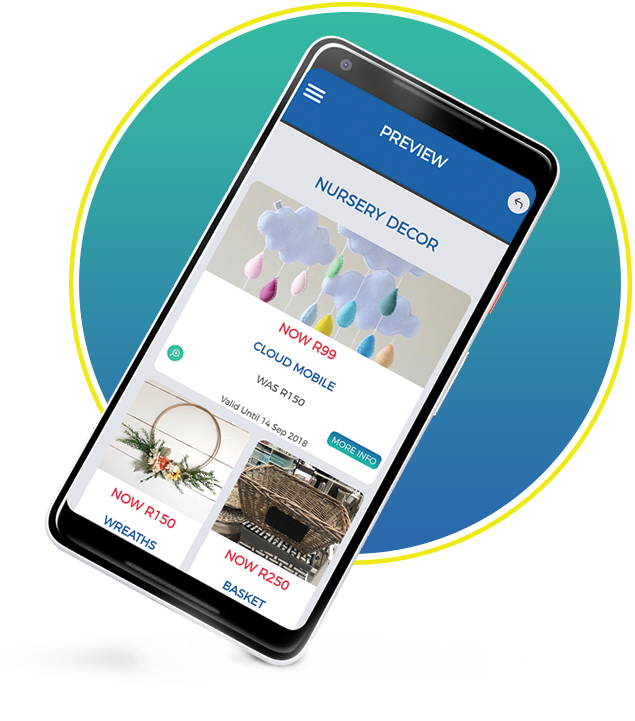In this vibrant image, a large yellow-outlined circle frames a gradient of blue and green hues, creating a visually appealing background. At the center of attention, a sleek black telephone is prominently featured. Above this centerpiece, there is a large blue rectangular box. This box contains three horizontal white lines, symbolizing a preview, alongside a white circle encasing a leftward-pointing arrow. The background of this box is light blue. 

Inside this blue box, an advertisement showcases nursery decor. It prominently features an image of a delicate mobile designed to hang over a baby's crib. The mobile consists of endearing little clouds and an array of colorful droplets in shades of blue, yellow, purple, and pink. In front of this image, a white box displays the text "Now R99" in striking pink font. Below this, it reads "Cloud Mobile, was R150," indicating a sale.

At the bottom left corner of the image, a small blue circle is present, while the bottom right corner hosts a blue button. An additional note informs viewers that the offer is valid until the 14th of September, 2018.

Additionally, there is a section with a floral decoration indicating further discounts: "Now R150 wreaths" and "Now R250 baskets." This section is accompanied by two relevant images to visually support these offers.